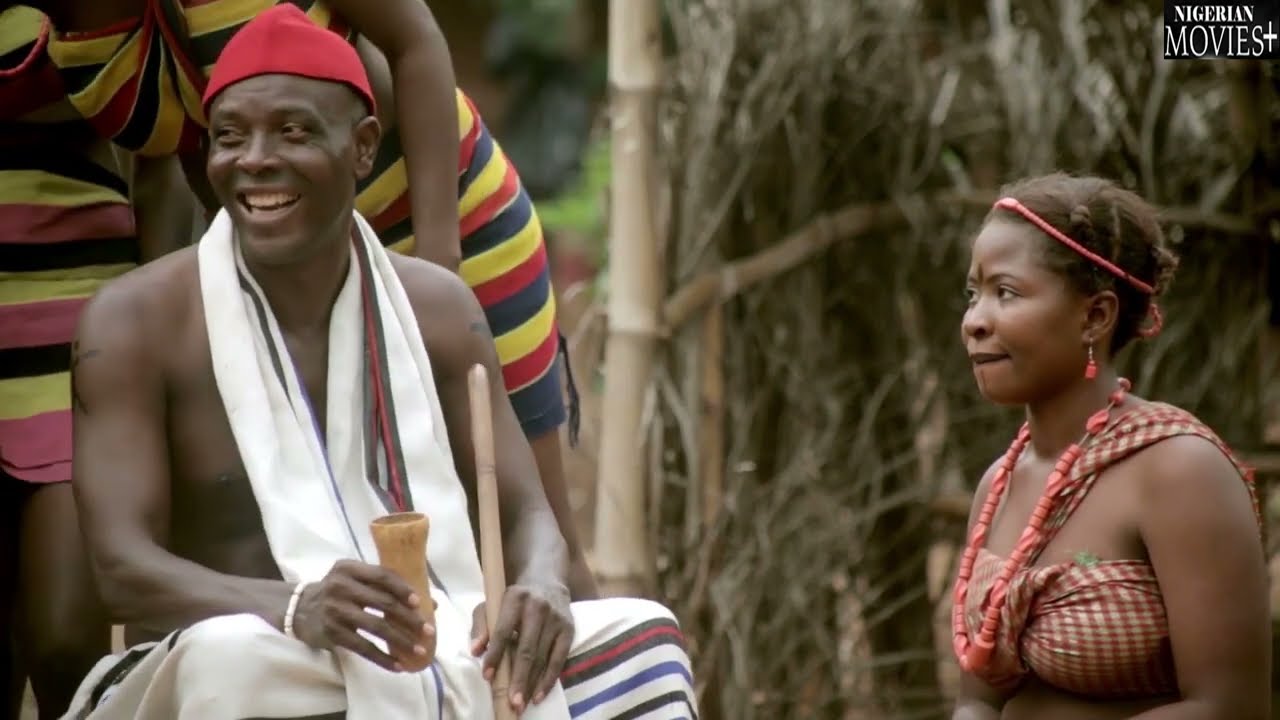In the image, a Nigerian couple, dressed in traditional tribal attire, stands out in a vibrant, native setting. Dominating the scene on the right is a young Nigerian woman with a serious expression. Her dark brown hair is tied back, adorned with a red beaded headband, while she wears matching red earrings and a red beaded necklace. Her outfit includes a red dress with a cross pattern, and she has a red dot on her forehead. Standing, she gazes at a shirtless man seated nearby. The man faces the camera with a smile, wearing a striped cloth around his neck and a red knit cap. He holds a thin wooden cup in his right hand and sports loose white pants adorned with red, black, and blue stripes. In the background, two women also dressed in colorful striped dresses can be seen. The upper right corner of the image contains a black rectangle with white text reading "Nigerian Movies Plus," suggesting a film or cultural context.